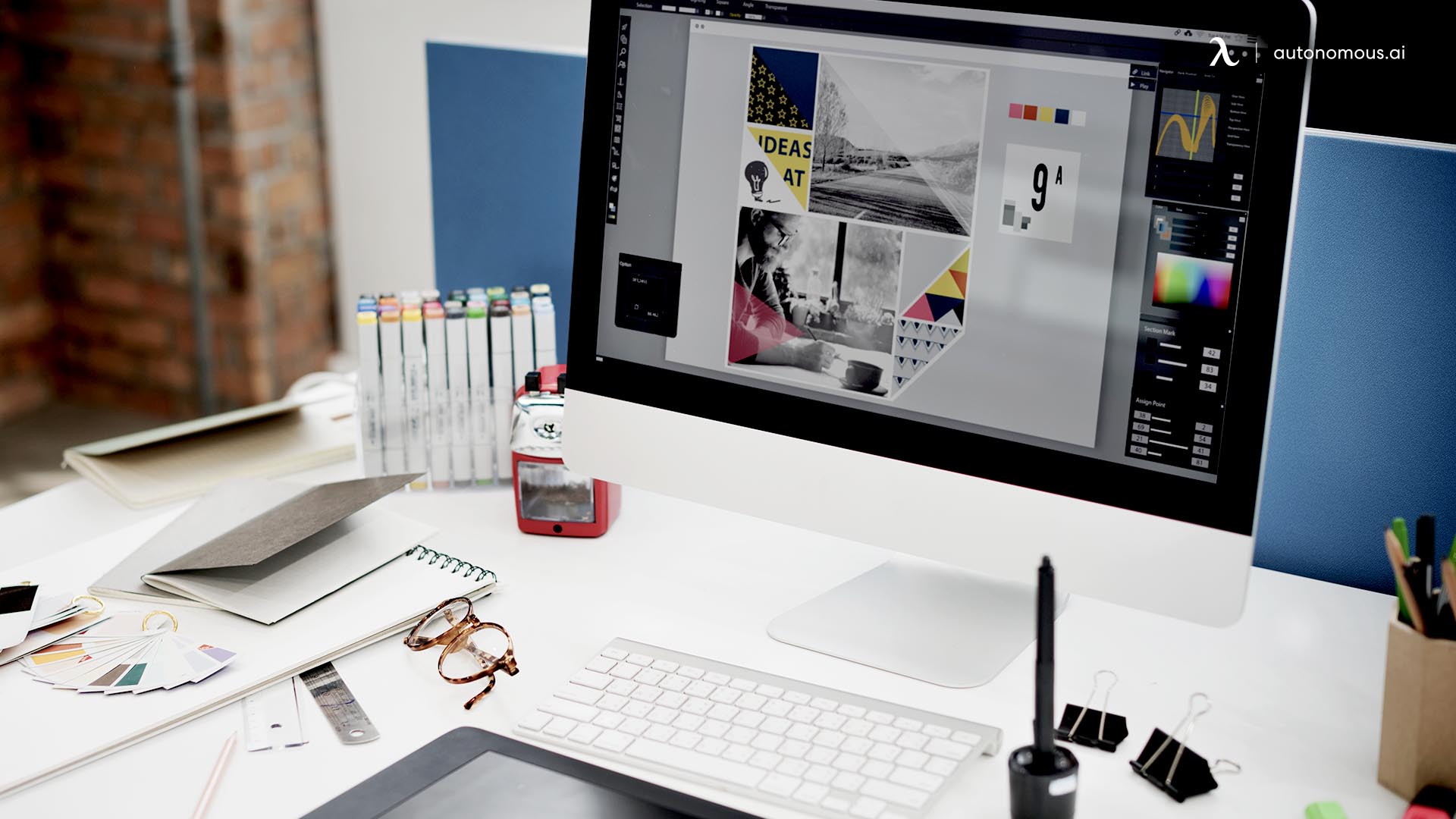The image depicts a U-shaped, white computer desk situated in front of a blue background, with a red brick wall blurred off to the right. Centered on the desk is a large monitor on a white stand, displaying graphic programs in the process of editing photographs. In front of the monitor sits a white keyboard, with a pair of tortoiseshell glasses resting to its right. The desk is organized with various tools, including a black pen in a plug-in base on the left, a tan octagonal pencil holder with various pens and pencils, a set of large black binder clips and paper clips, and a box of color-coded graphic markers in a Lucite holder. Scattered around the workspace are several rulers, pencils, a red rubber stamp, paint swatches, and a couple of open books, including a brown-covered book and an open sketchbook. In the upper left side of the image, the text "Autonomous.ai" is visible. The overall scene is well-lit and professionally arranged, emphasizing the creative and technical environment suitable for someone in the graphic design industry.